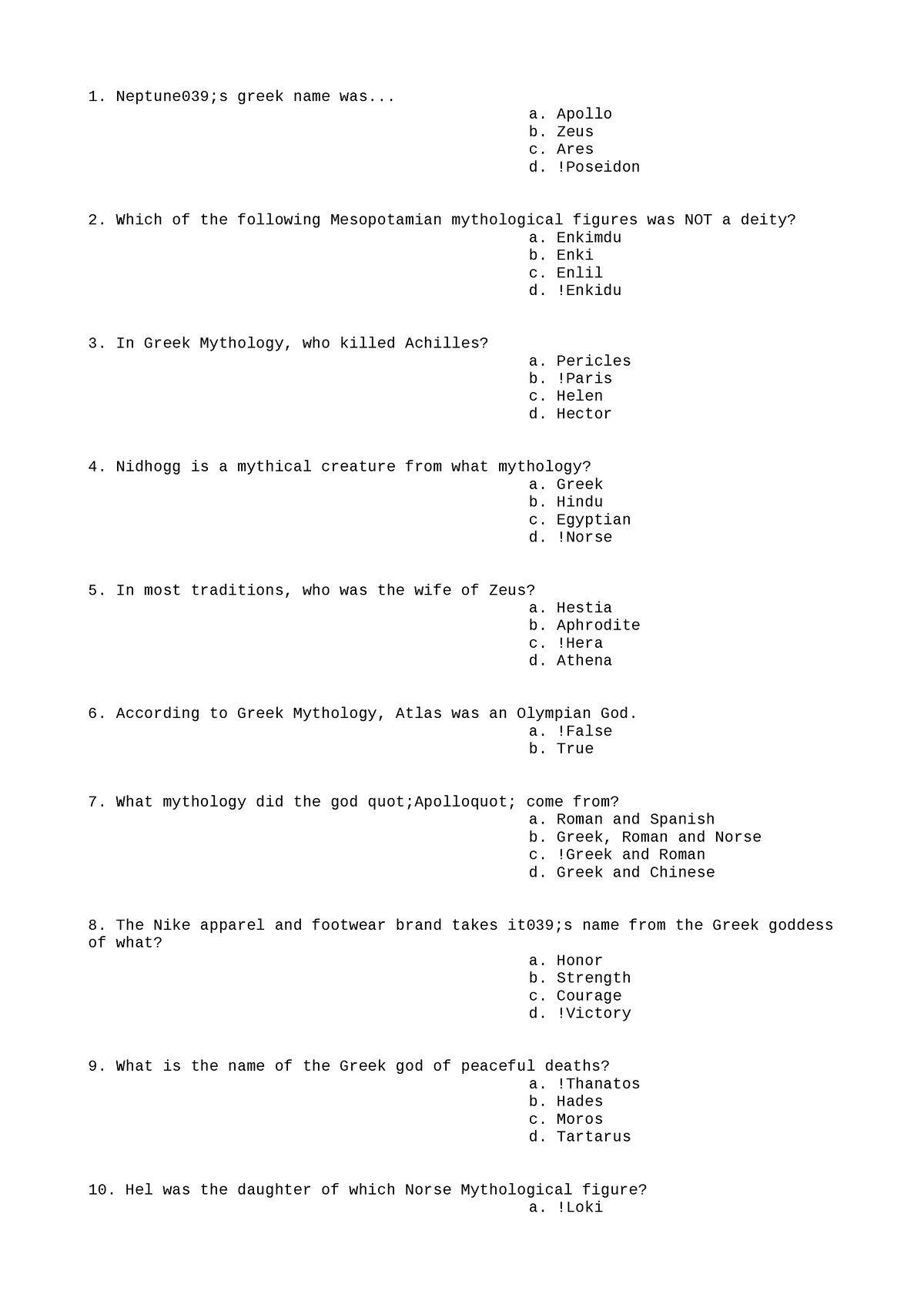The image depicts a black-and-white webpage resembling a question-and-answer format. The layout is reminiscent of a quiz or test, featuring a series of ten questions, each accompanied by four possible answers labeled A, B, C, and D. For instance, one of the questions reads: “Nepanese 39, a Greek name was,” followed by the choices Apollo, Zeus, Aries, and Poseidon. Another question asks, “In most traditions, who was the wife of Zeus?” with the options being Aphrodite, Athena, Hestia, and Hera. Notably, the image appears to be cut off at the last question, only showing option A without the possible B, C, or D answers. The page lacks any headings, instructional text, or contextual information to indicate its purpose or source, leaving the user with just the raw questions and answer choices.